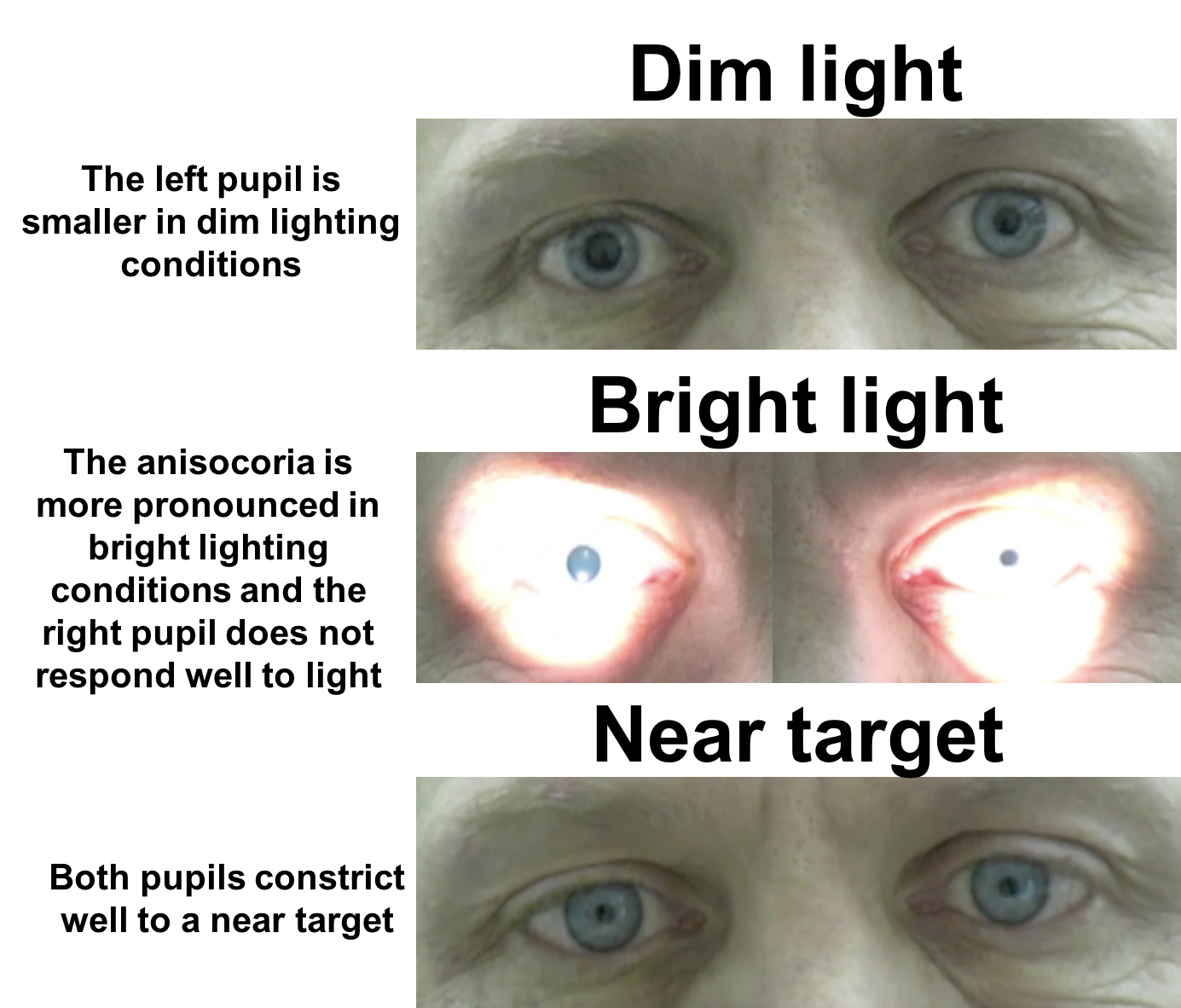The image is a triptych of a man's face, showcasing the responses of his blue eyes under different lighting conditions for educational or clinical analysis. The top section, labeled "dim light," highlights that the left pupil is smaller in low lighting conditions, revealing anisocoria where one pupil is larger than the other. The middle section, designated "bright light," indicates that the anisocoria becomes more pronounced, with the right pupil not responding well to light exposure. The bottom section, marked "near target," shows both pupils constricting equally when focusing on a nearby object. This detailed visual analysis appears aimed at understanding pupil reactions to various stimuli, likely for educational or medical purposes, and features the same set of older, clearly blue eyes in each segment.